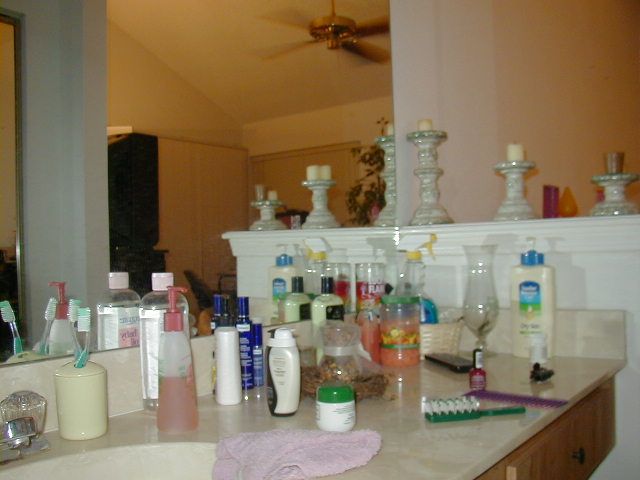A rectangular photograph captures a tidy bathroom counter in sharp detail. Dominating the top left quarter of the image is a large bathroom mirror that spans the wall behind the counter, reflecting the pristine and orderly bathroom. Within the mirror's reflection, the room's white-painted walls and a ceiling fan draw attention. The fan, set into motion, appears blurred but reveals its five-blade design with a brown brass base and a slender brass-colored pole.

The counter itself is a smooth surface with a tannish-gray hue. In the bottom left corner of the image, a built-in sink basin is visible, featuring a small silver-colored faucet paired with a clear plastic knob. Adjacent to the faucet, a porcelain ivory white toothbrush holder stands, elegantly designed as a cup with a lid punctuated by small holes. Two identical toothbrushes are neatly inserted into the holder, maintaining the overall neat and organized aesthetic of the bathroom.